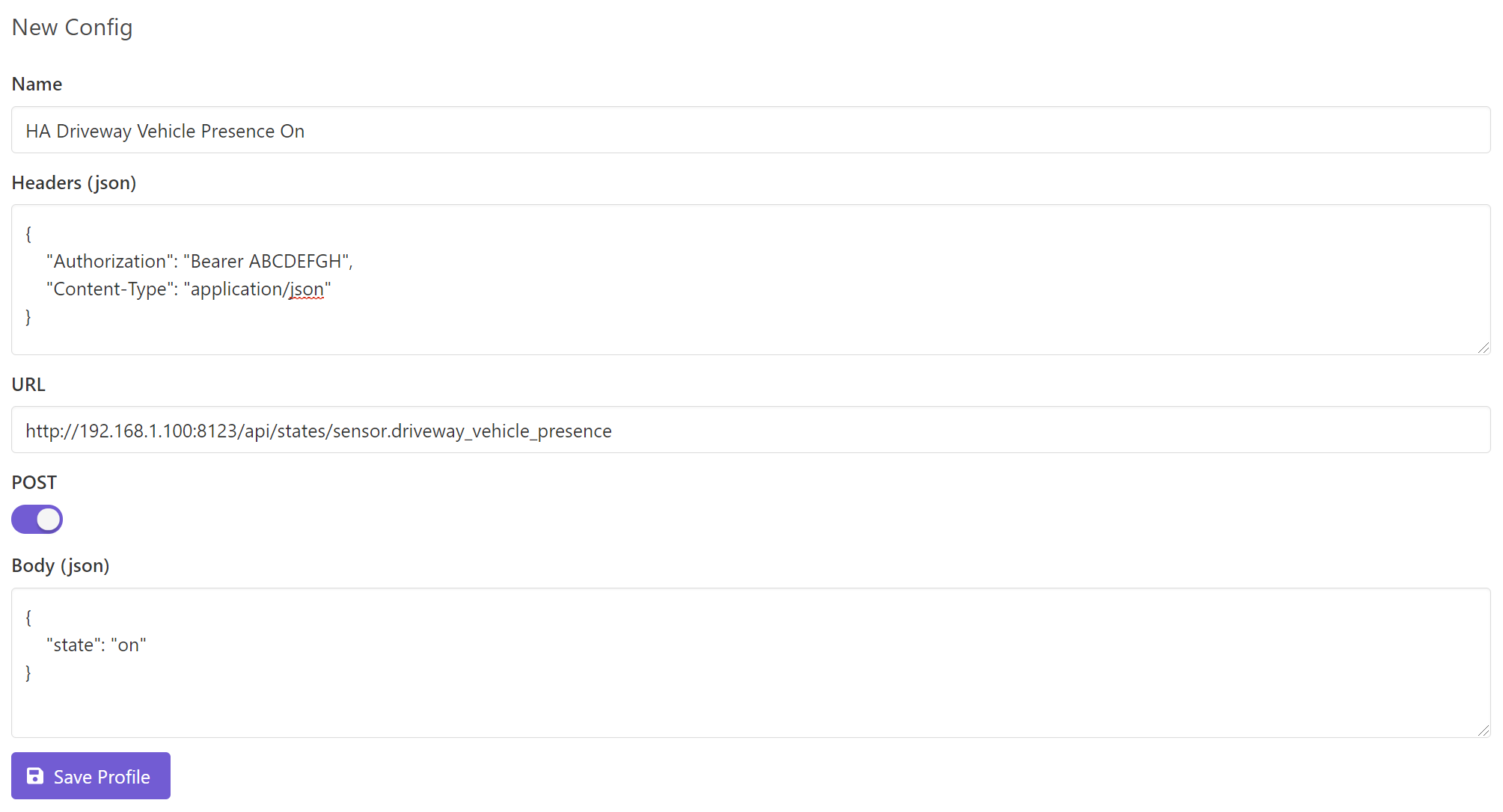This screenshot depicts a settings pop-up on a computer interface. The background is predominantly white, particularly noticeable at the top left. At the top, there is thin gray text that reads "New Config." Below this, aligned to the left, there is smaller bold, dark gray text that reads "Name." Directly beneath this, there is a white text entry box with a thin light gray outline, containing the black text "HA driveway vehicle presence on."

Following this, there is another piece of bold, dark gray text that reads "Headers (JSON)." Under this heading, there is a large text entry box bordered by curly brackets on the top and bottom. Inside this box, two lines of gray text are enclosed in quotes: the first line reads "Authorization: 'Bearer ABCDEFGH'", and the second line reads "'Content-Type': 'application/json'". On the bottom right corner of this text box, two dark gray lines are rotated 45 degrees, possibly indicating a code formatting feature or a graphical element.

Beneath this section is another bold, dark gray header labeled "URL." Under this label, there is a single-line text entry box containing the URL "http://192.168.1.100:8123/api/state/sensor.driveway_vehicle_presence".

The final section features a bold, dark gray header labeled "Post." Directly below this, there is a purple selection button with a white circle positioned on its right side, indicating a toggle or selection option within the interface.